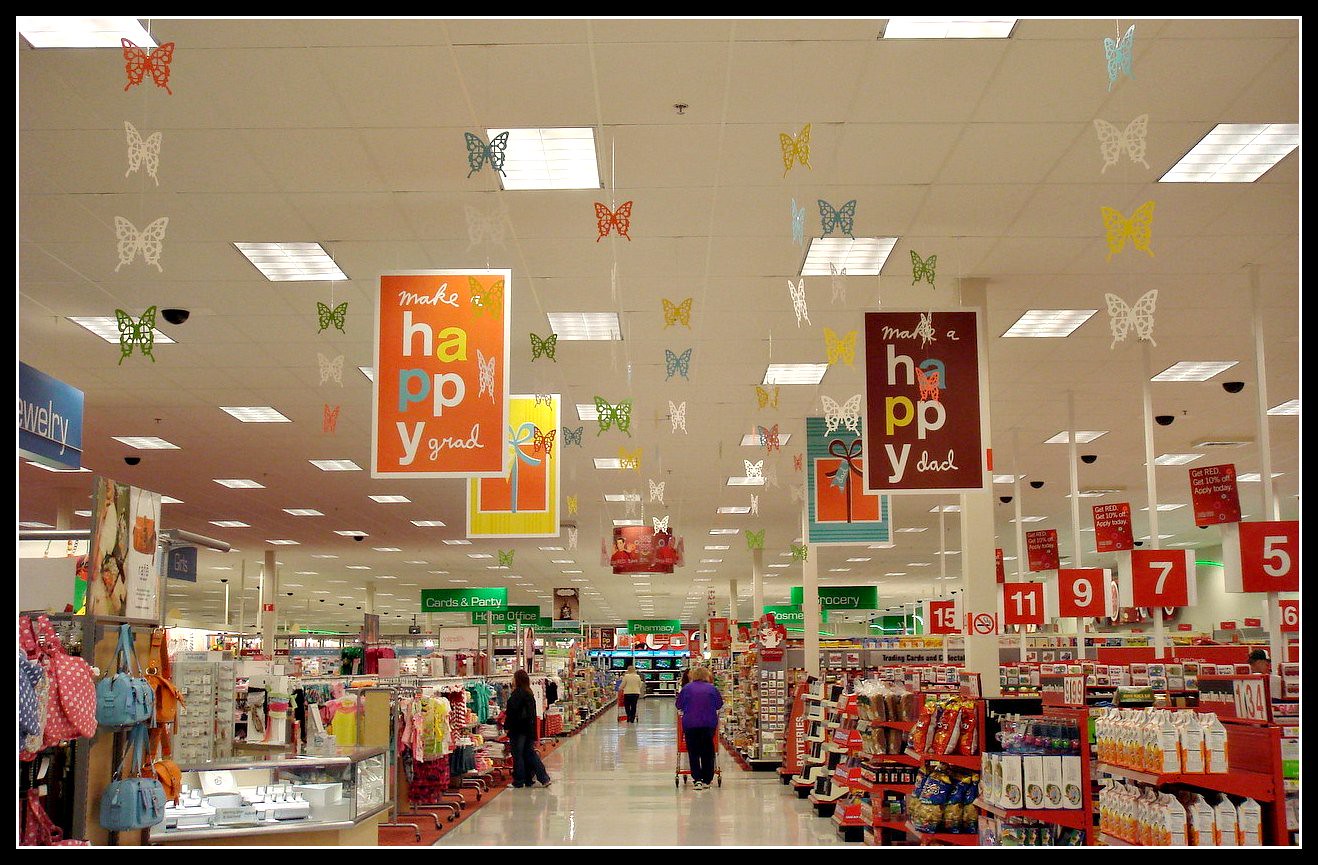The horizontally rectangular image, framed with a thin black border, captures the bustling interior of a retail store. Central to the composition is a wide, spacious aisle leading towards the back of the store, where a few shoppers, seen from behind, push their carts leisurely down the lane. On either side of this central aisle, several horizontal aisles branch off, each marked with red signs displaying aisle numbers in white, organized sequentially from lowest to highest. Dominating the upper part of the scene, large, clean white columns rise to meet a tile ceiling interspersed with fluorescent lights that cast a bright, even illumination throughout the store. Suspended from the ceiling are whimsical butterfly figures, adding a touch of playful decor to the otherwise practical setting.